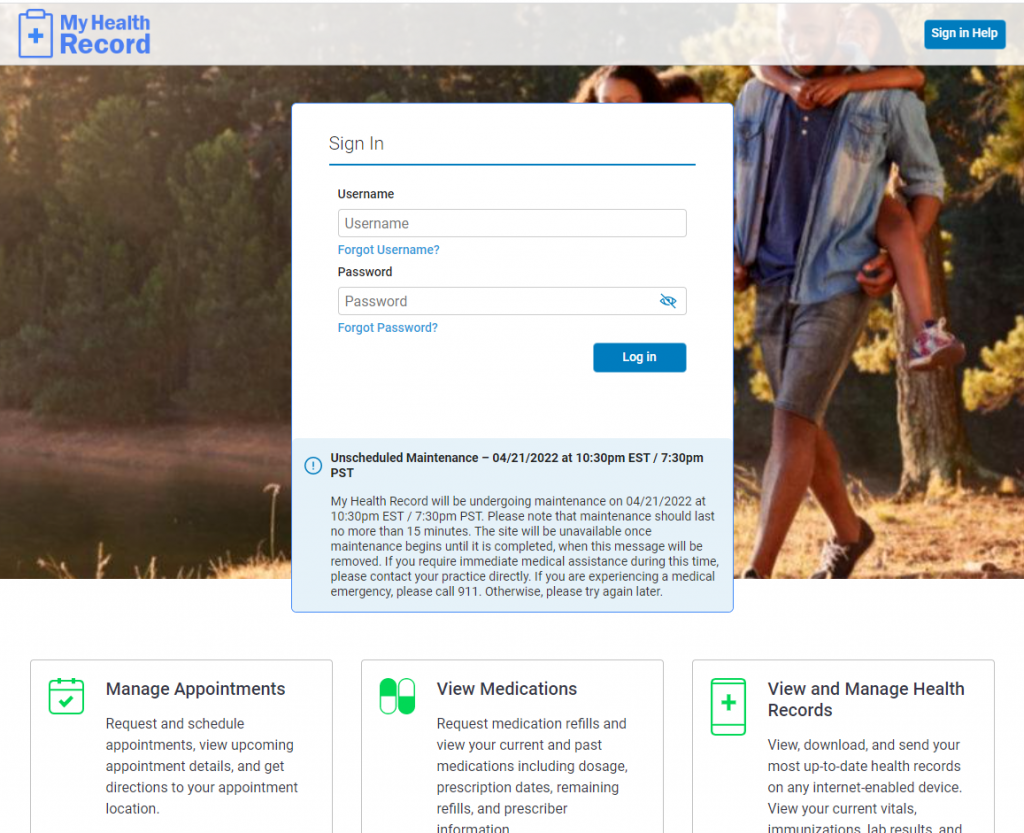The image captures a screenshot of the My Health Record website, a platform designed for users to access their medical records. In the top left corner of the navigation bar, the site name "My Health Record" is displayed in blue, likely clickable. On the far right of the navigation bar, options for signing in or seeking help are prominently featured. The central focus of the page is the login section, prompting users to enter their username. If forgotten, a blue text link offers username recovery. Below, a similar setup exists for password entry and recovery, complemented by the recognizable blue eye icon for toggling password visibility. After entering their credentials, users can proceed by clicking the blue "Login" button.

A banner across the page informs users of scheduled maintenance on 4-21-2022 from 10:30 PM to 7:30 PM PST, indicating potential login disruption during these hours.

Beneath the login section, three main functionalities are presented:
1. **Manage Appointments**: Accompanied by a green icon with black text, this option allows users to schedule medical appointments.
2. **View Medications**: Represented by a green icon resembling joined pills, this section enables users to review their current medications.
3. **View and Manage Records**: With a large green square icon, this feature grants access to past medical records and health information.

Overall, the My Health Record website serves as a comprehensive tool for managing various aspects of one's medical history, though the screenshot doesn't specify the affiliated health organization.